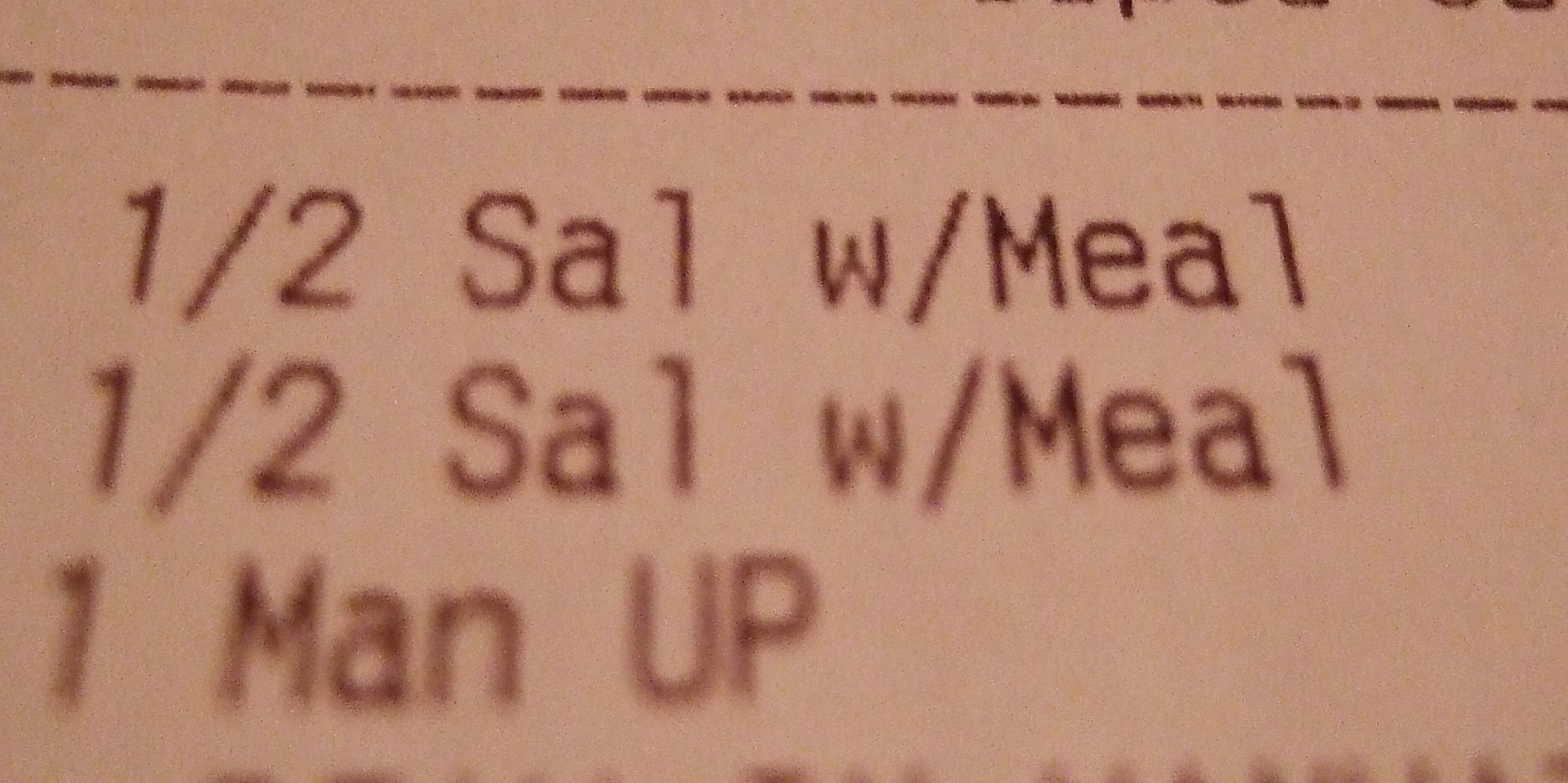The image features a close-up view of a pinkish-brown receipt, tilted upwards and zoomed in to reveal limited details. At the very top, there's a border of purple-brown lines or etches, which are partially visible on the upper right side. Below that, a perforated line runs horizontally across the image. The receipt's text, appearing in a dark shade of brown or black, reads "1/2 SAL W/ MEAL," repeated on two lines. At the bottom left, the text "1 MAN UP" stands out, with 'UP' in capital letters.